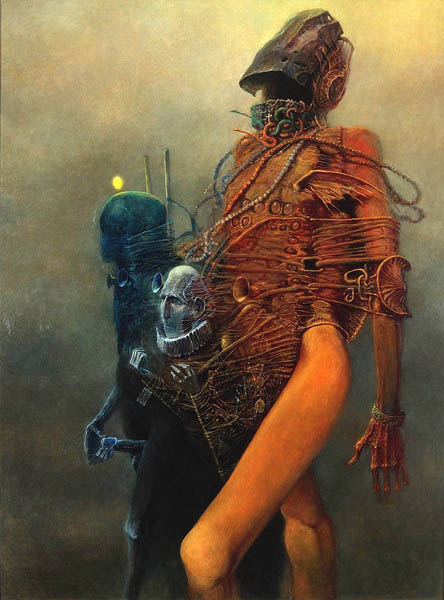The image is a highly detailed, dystopian, fantasy painting set in a dark, misty, and gray outdoor scene. It features three humanoid creatures walking together. The figure closest to us is tall and skeletal with long bare legs and arms thin like bones. This character's head is enveloped in an open yet seemingly hollow armored mask, making it appear almost lifeless. It has chains wrapped around its body and a disembodied skull hanging from it, lending a haunted, cyborg-like appearance. Next to this eerie figure is a shorter old man with enormous ears, clad in a black robe with a white collar, and holding his hands out in front of him. To his side walks another humanoid, slightly shorter than the first but taller than the old man. This character is entirely encased in black armor with a masked helmet, adding to the surreal and disturbing ambiance of the artwork. The overall scene seems to combine elements of science fiction and horror to create a grim, futuristic tableau.